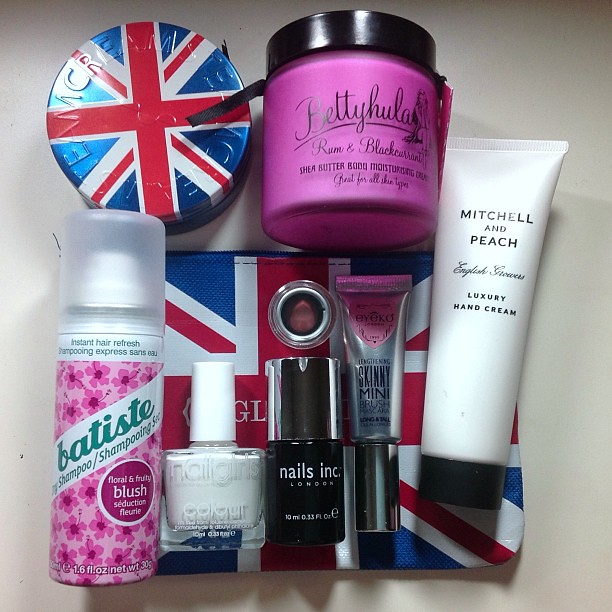The image displays an assortment of beauty products arranged on a makeup bag themed with the British flag. At the top left, there is a circular tin adorned with the British flag. Next to it, there is a small jar featuring a black lid and metallic purple bottom. This jar is labeled "Betty Hoola Shea Butter Body Moisturizer" and is great for all skin types. On the right side of the image, a white tube of Mitchell & Peach Luxury Hand Cream is noticeable. Below these items, atop the makeup bag, is a collection of various nail polishes and tubes: a thin spray bottle labeled "Batiste," a small white vial of nail polish with a white cap, a black nail polish with a silver cap, and a tube marked "Skinny Mini." The meticulous arrangement of these colorful and varied beauty items creates a visually appealing display of cosmetic essentials.